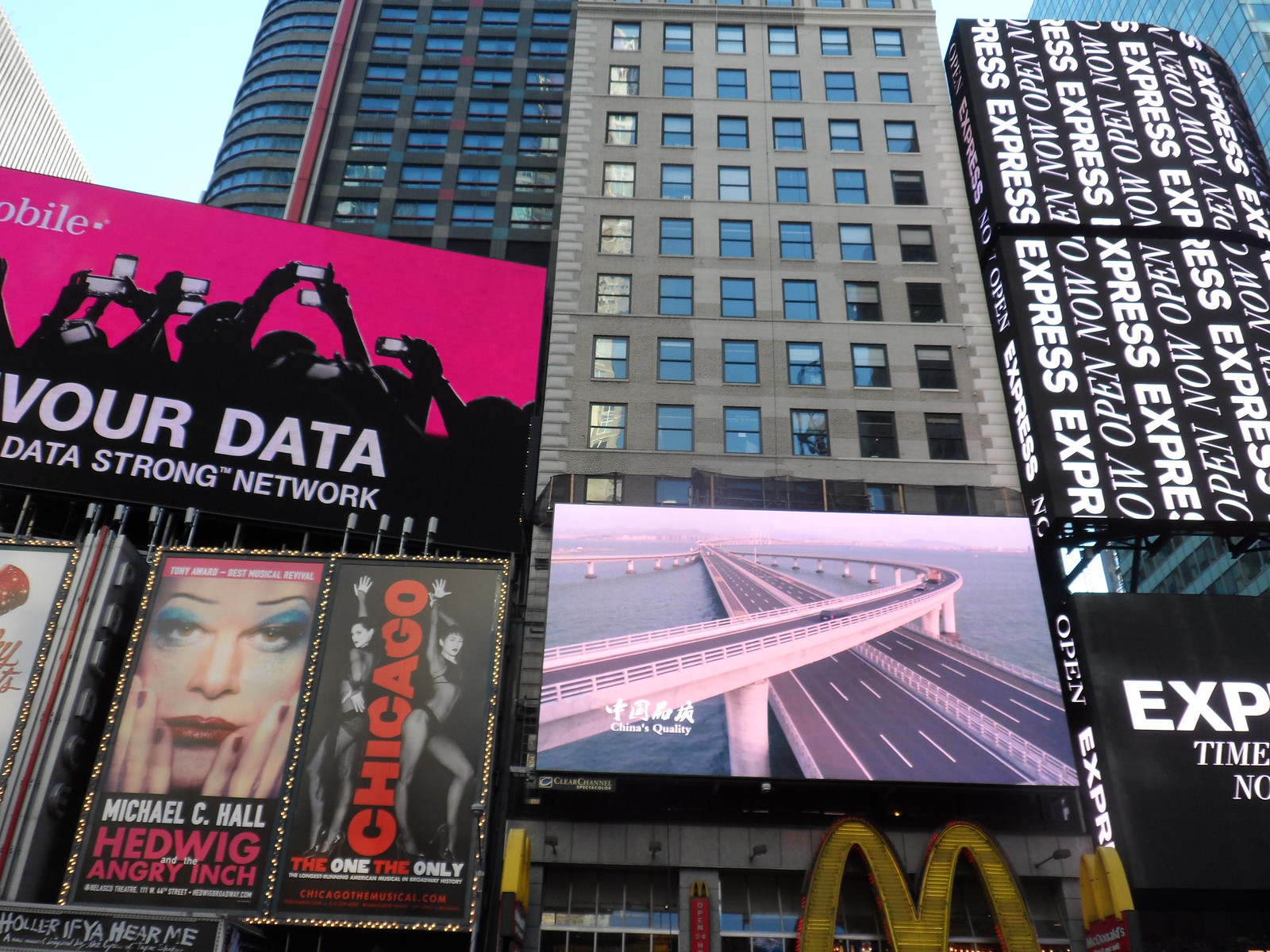This photograph, taken in Times Square, captures an urban landscape teeming with advertisements and multi-story buildings. Centered in the image, a large electronic billboard displays an image of a double bridge over water with Asian writing that reads "China's quality." To the left, there are multiple advertisements, including one for the play "Chicago" and another featuring Michael C. Hall in "Hedwig and the Angry Inch." Above these, a T-Mobile billboard stands out with its pink and black graphics, showcasing people holding up phones and the tagline "Your data, Data Strong Network." At street level, a McDonald's sign is visible at the bottom edge. Above it, another screen shows a highway and bridge image. Dominating the right side, a slender building has a sign for "Express, Open Now." A prominent multi-story gray building with numerous windows rises above the advertisements, and on the far left, a curved building corner with many windows is also visible. The image intricately displays both the architectural variety and the vibrant commercial activity characteristic of Times Square.